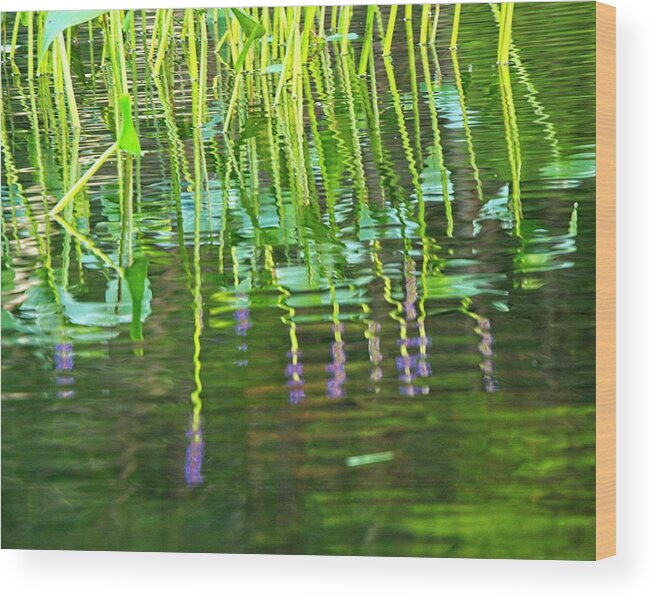The image depicts a serene scene of a pond or lake, where the primary focus is on the reflection of aquatic plants in the water. In the upper left-hand corner, light green stems with a few dark green leaves extend from the water's surface. At the tops of these straight, reed-like stalks, there are clusters of lavender-purple flowers. The reflection of these flowers and stems is beautifully captured in the water, adding a captivating visual element where the ripples give the illusion of curly stems. The body of water itself has a greenish tint, enhancing the natural palette. The painting appears to be done on a thick block of wood, as evidenced by its visible sides, suggesting a handcrafted, rustic feel. The overall colors in the artwork are dark greens, light greens, and the striking purple of the flowers, set against the tranquil backdrop of the pond or lake on a presumably sunny day.